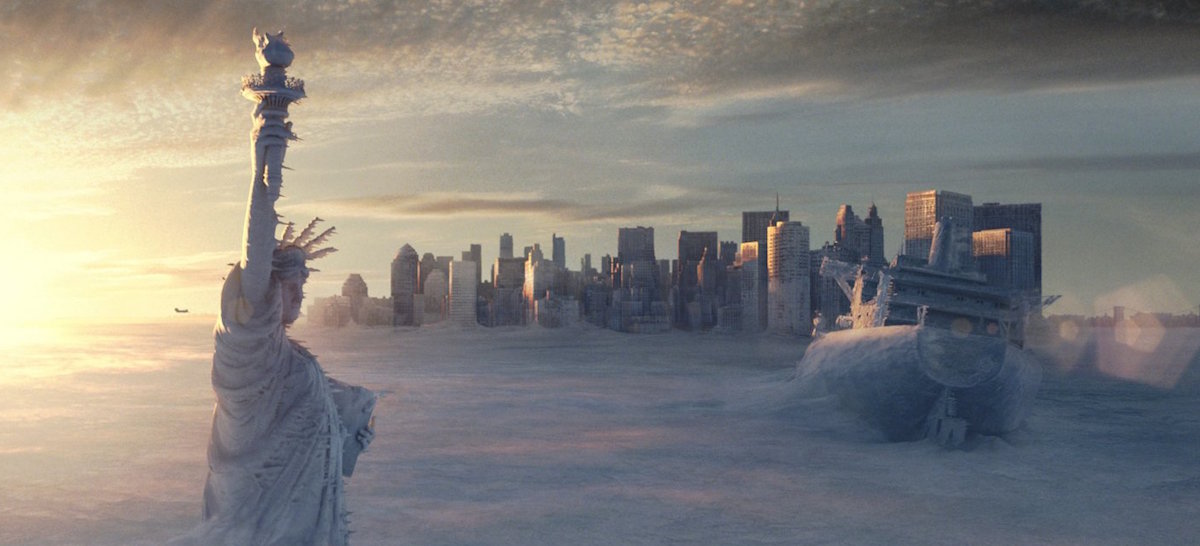This panoramic 3D rendering showcases a captivating ethereal and fantastical vision of the future. On the left side, the iconic Statue of Liberty stands proudly in the foreground, meticulously detailed and illuminated. To the right, a steampunk-inspired ship gracefully hovers above the water, exuding an aura of mechanical ingenuity with its brass fittings and intricate design. The backdrop features a densely populated cityscape, teeming with towering skyscrapers that define a futuristic New York City skyline. Puffs of clouds float in the sky, adding depth and dimension to the scene. In the distant background, an airplane soars high, just to the left of the Statue of Liberty, hinting at the fusion of old and new worlds in this imagined future.